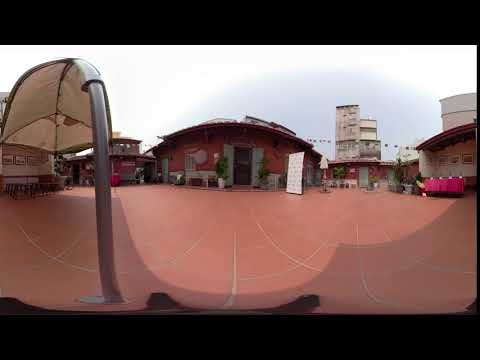The image depicts a spacious courtyard-like area surrounded by short, reddish-burgundy, one-story buildings. These structures have a distinct vintage look, with one prominent rectangular building standing at the center, featuring a black door and green shutters on either side. Adjacent to this building on the right, there is a white sign and possibly a table set outside. The ground of the courtyard is covered in square, red brick-like tiles, suggesting a walking space for people. On the left side, a pole with an umbrella attachment offers shade, tapering off in a teardrop shape. In the background, an old, gray concrete skyscraper, likely seven to eight stories high, towers above the smaller buildings, set against a sky that transitions from a faint blue to white near the buildings. There's also a smaller structure of similar color to the left of the central building. The image has a warped, fisheye effect, which curves and distorts the scene, enhancing the historical, almost village-like ambiance.